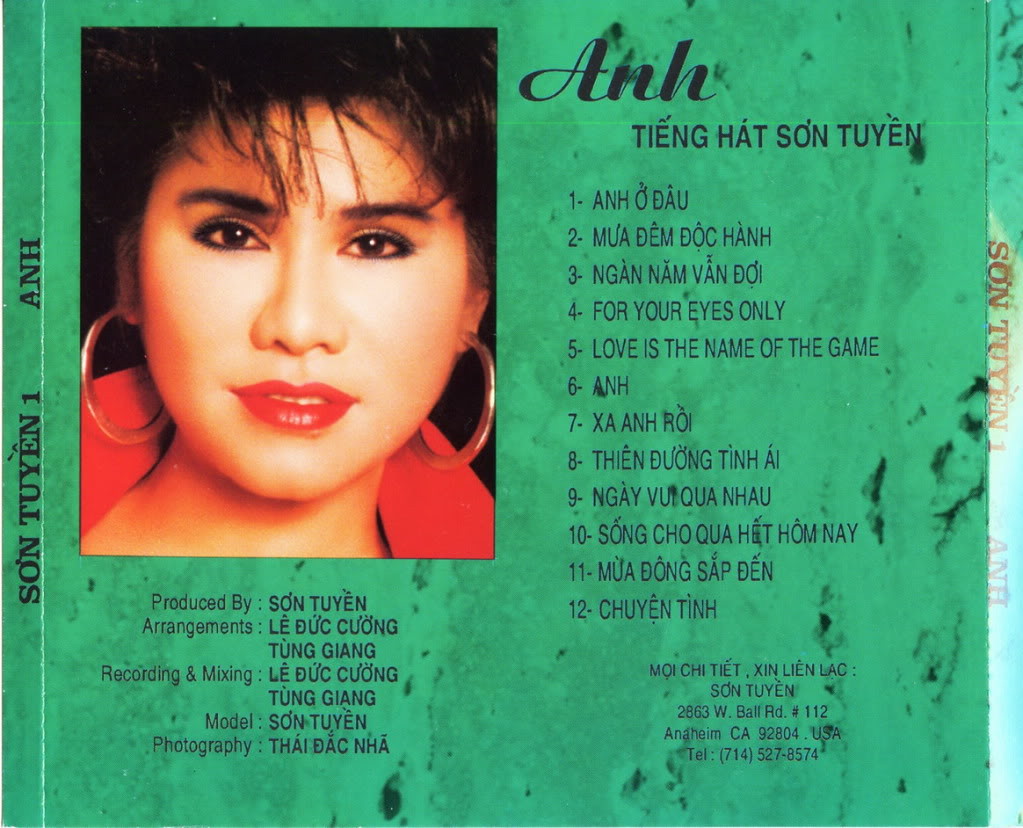The image is a green album cover that prominently features a Vietnamese singer named Anh. In the upper left corner is a close-up picture of Anh, a woman with black hair, bangs, black eyebrows, brown eyes, and red lips. She wears a striking red coat with a tall collar and large circular silver earrings. The background behind her portrait is black. 

To the right of the image is the album title "ANH," followed by a list of songs numbered from 1 to 12, written possibly in Vietnamese. Below her picture, in the bottom left corner, are the production credits: produced by Tsong Tuyen with arrangements by Le Duc Quang and Tung Giang, and recording and mixing by Le Duc Quang and Tung Giang. Photography credits go to Thai Doc Nha. The bottom right corner contains some contact information. This detailed composition suggests that this is indeed the cover of a Vietnamese singer's album.